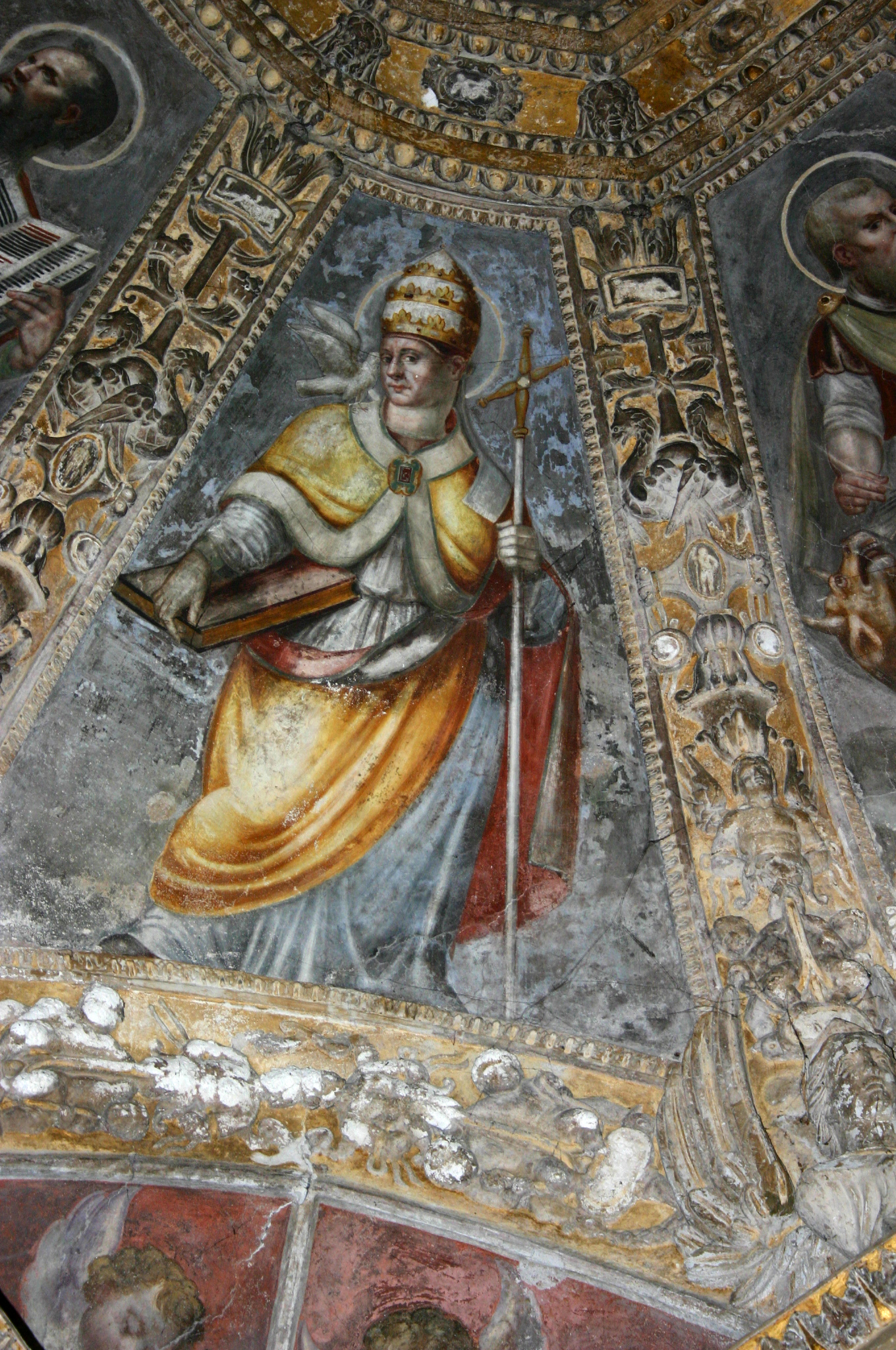The image depicts a close-up of a highly ornate and spectacular old artwork painted on the ceiling, likely within a church or chapel. The focal point of the painting is a religious figure, dressed in a long white robe with yellow accents, adorned with an orange and yellow cloak, and a red and white sash. The figure has fair skin and wears a distinct, ornate headdress, gold and white in color, which is acorn-shaped and decorated with intricate patterns. In his left hand, he is holding a large, faded reddish-brown book with gold embellishments, and in his right hand, he carries a white staff topped with a gold cross. Surrounding this central figure are elaborate gold, brown, and silver adornments, forming a decorative border. The painting is part of a larger scene featuring multiple figures, with others partially visible but not the focus of this image.